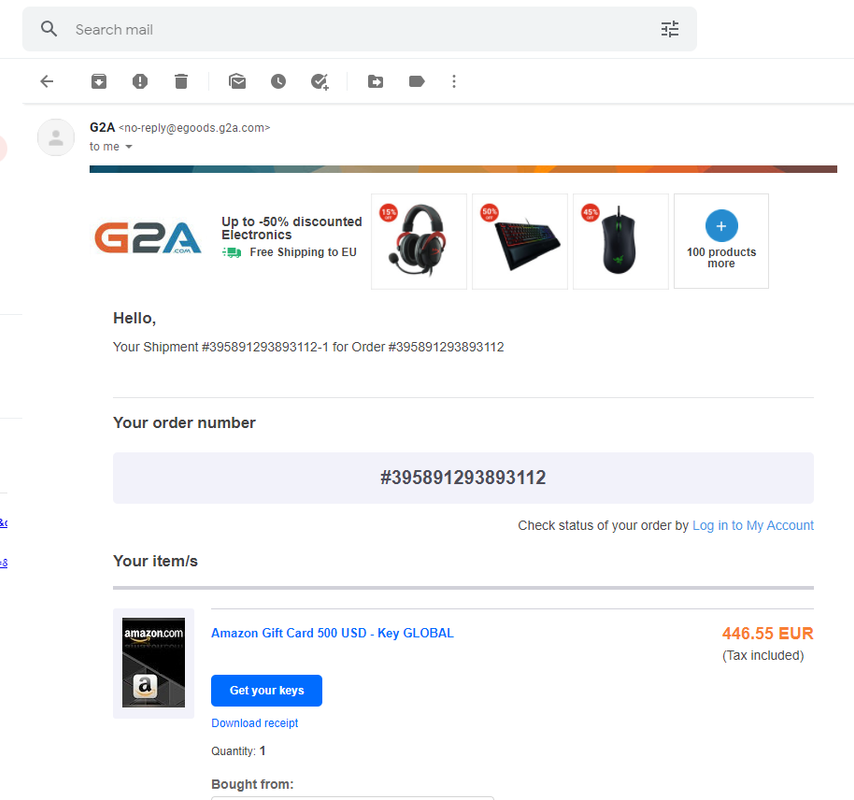This is a detailed screenshot displaying an email received from G2A, with the sender's address listed as noreplyategoods.g2a.com. The email contains an invoice and an order confirmation featuring an order number: 395891293893112. 

The primary content of this order is an Amazon gift card valued at $500 USD. The gift card image showcases it in a sleek black case, and the URL blackcasecaseamazon.com is mentioned. There is a prominent blue button labeled "Get Your Keys" and another option for "Download Receipt," also in blue. The quantity ordered is 1, and the total cost is specified as 446.55 Euros, marked in bold orange text. 

The webpage background is white. An additional shipping number is noted: 39581293893112-1. 

At the top of the email, there is a banner from G2A announcing "Up to -50% Discounted Electronics & Free Shipping to the EU." Additional visuals include images of office items: a headset, a keyboard, and a computer mouse.